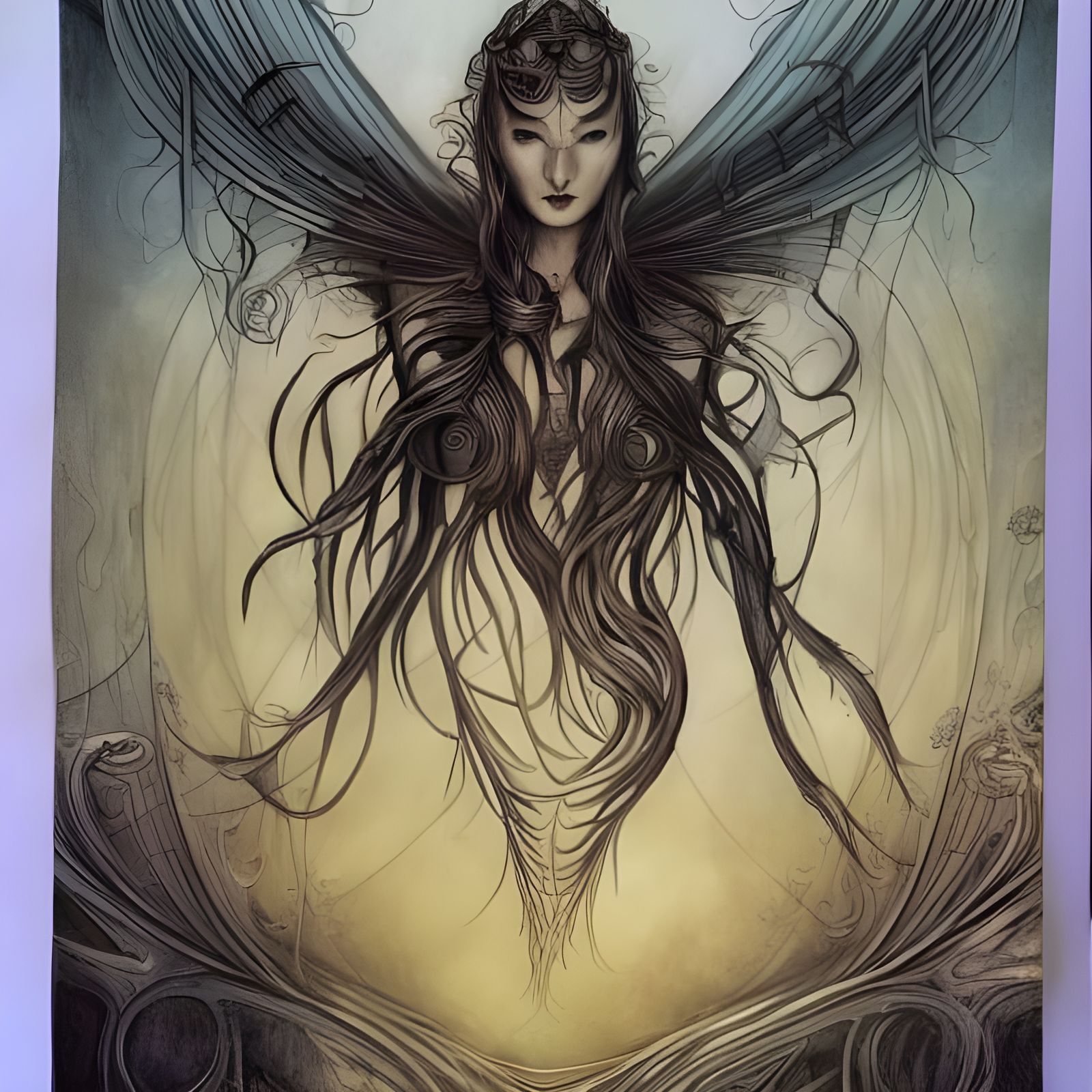The image depicts a fantastical, ethereal woman drawn in a graphic style with an emphasis on light blue, tan, and brown shades. Her body is not distinctly defined, appearing as if she's floating, with only her head, a portion of her chest, and an impression of a dress formed by her cascading, dark hair. The hair flows down her body and circles her chest, merging seamlessly with the dress-like structure, leaving the distinction between hair and attire ambiguous. Her face, which has a light complexion and distinctly oriental features, is adorned with interesting upward-curving eyebrows. From just behind her neck, two dark wings protrude, enhancing her mythical, almost creature-like appearance. The image has strand-like trims surrounding it, contributing to its fantasy atmosphere, and the background remains simple and unembellished. The woman's appearance is accentuated by her dark hair and black lips, contributing to the overall otherworldly aesthetic.